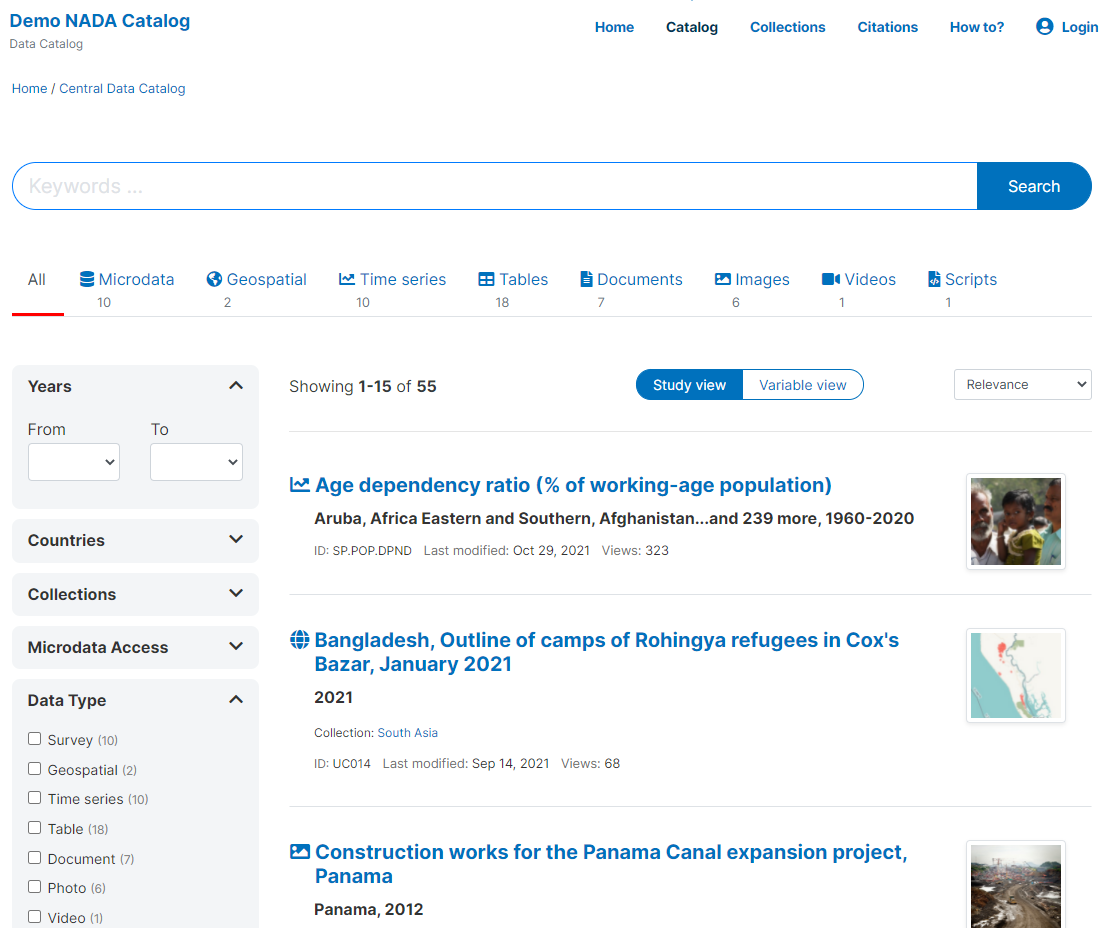Screenshot of a website with a white background. At the top, there is blue text reading "Demo NADA Catalog" (N-A-D-A), followed by darker gray text that says "Data Catalog." Below this is a smaller line of blue text that reads "Home" and, in smaller print, "Home / Data / Central Data Catalog." 

Moving horizontally to the right, the menu options include "Home," "Catalog," "Collections," "Citations," "How-to?" and "Login," where "Catalog" is in darker print and the others are in blue.

Below the menu, there is a search bar with the placeholder text "Keywords." Underneath the search bar, a set of navigation tabs is arranged horizontally: "All," "Microdata," "Geospatial," "Time Series," "Tables," "Documents," "Images," "Videos," and "Scripts," with "All" being underlined in red.

To the left, there is a gray sidebar labeled "Years" with input fields for "From" and "To." Additional filters include "Countries," "Collections," "Microdata Access," and "Data Type," each with a corresponding drop-down menu.

In the main content area, it says "Showing 1 of 15 of 55," and there are two view options: "Study View" with a blue background and white text, and "Variable View."

Listed studies include:
- "Age Dependency Ratio, Bangladesh"
- "Outline of Camps of Rohingya Refugees in Cox's Bazar, January 2021"
- "Construction Works for the Panama Canal Expansion Project, Panama"